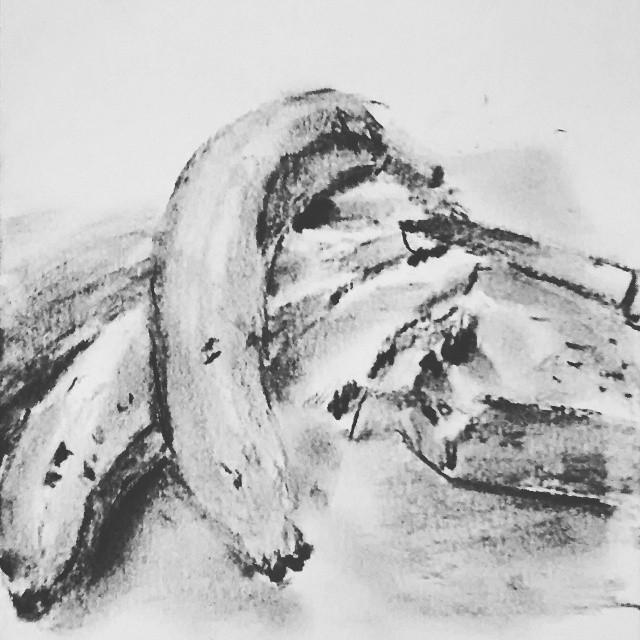This square-shaped, black and white image appears to be a low-resolution and blurry sketch. It gives an impression of a charcoal or graphite drawing, poorly rendered and abstract in its form. On the upper part of the image, the background is primarily white, transitioning into a mix of lighter and darker shades of gray and black towards the bottom. The focal point of this image seems to be long items, presumably bananas, with at least three distinctly visible on the left side. These objects have a downward flow and are detailed with varying shades to give them dimension. The right side of the image remains ambiguous, containing only indistinct black splotches and white areas, making it difficult to decipher any specific elements. Overall, this image’s combination of abstract sketching and low quality make it challenging to interpret clearly.